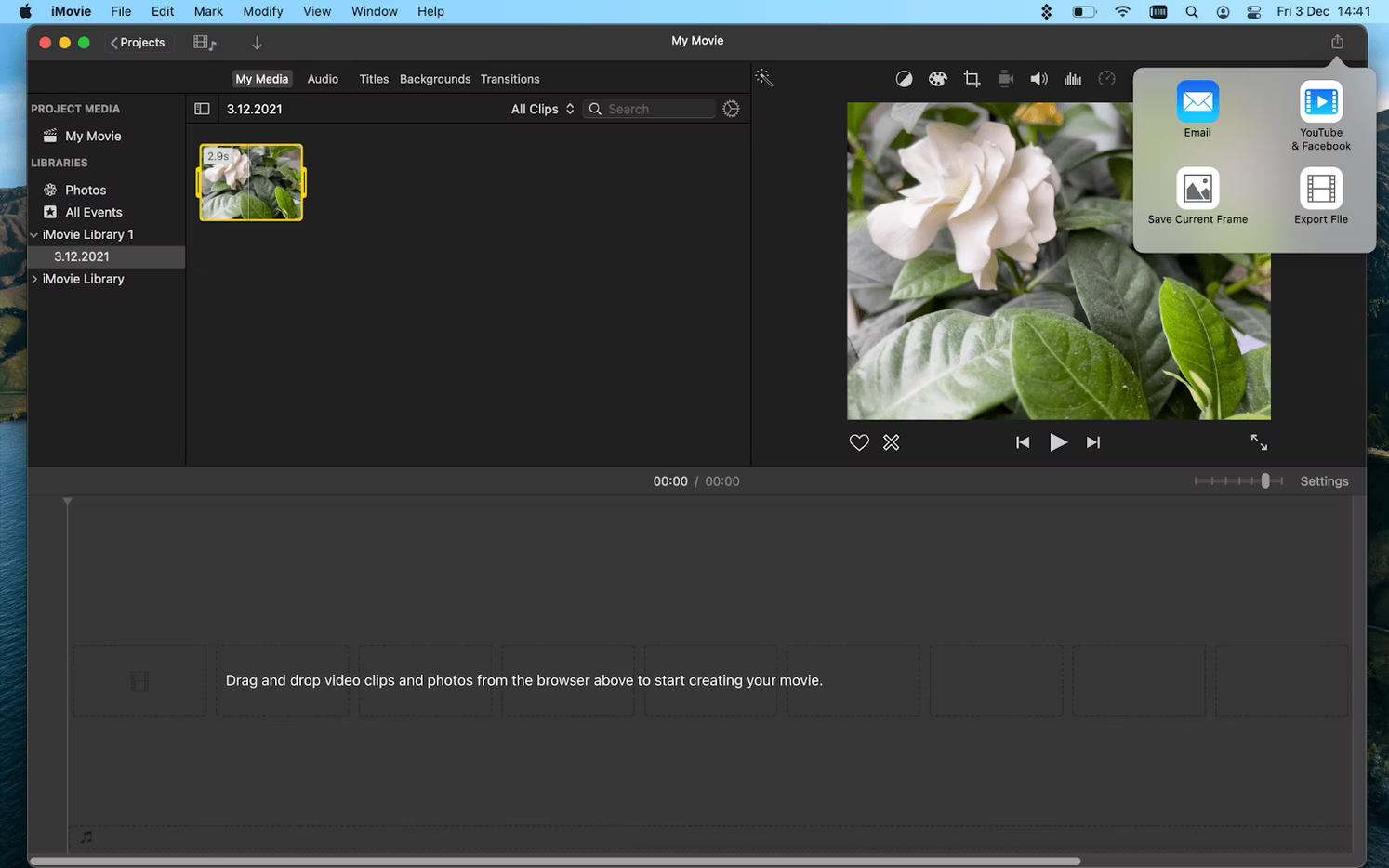This screenshot captures a detailed view of the iMovie interface on an Apple computer. At the very top of the screen, the menu bar lists options: iMovie, File, Edit, Mark, Modify, View, Window, and Help. To the right, additional system icons are visible alongside the date, Friday, December 3rd, 1441.

The iMovie interface is prominently displayed, indicating that a project is either being edited or ready to be played. A message at the bottom of the screen instructs users to "drag and drop video clips and photos from the browser above to start creating your movie."

In the upper left corner, the panel is labeled "Project Media 3.3.12.2021," showing various library sections: iMovie with its icon, Libraries, Photos, All Events, iMovie Library 1.3.12.2021, and iMovie Library.

A selected image of a white flower with green leaves and subtle yellow highlights is shown twice: once as a small preview box and again as a larger, more detailed display. Below this, playback controls are present, featuring buttons for play, rewind, fast forward, and enlarge, along with a heart icon and an X icon. The timing indicator reads 00:00/00:00, suggesting no video has been played yet.